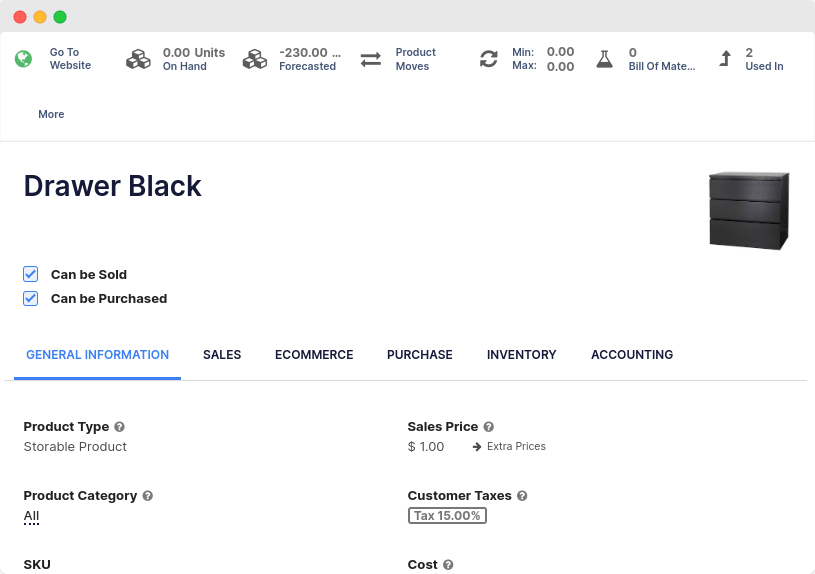A detailed image caption could be:

"The image depicts a management interface screen for an inventory tracking system, focusing on a product categorized as a 'storable product' which is a black dresser with three drawers. Key information shown includes: '0.00 units on hand' and a 'forecasted' value of '-230,' indicating a shortage or future demand mismatch for the product. The options 'can be sold' and 'can be purchased' are both checked, affirming the product’s eligibility for sales and purchases. The highlighted tab is 'General Information,' displayed in blue, while other sections like 'Sales,' 'E-commerce,' 'Purchase,' 'Inventory,' and 'Accounting' remain unselected in white. Additional details include a 'product type' marked with a gray circle and a white question mark, indicating it might need defining. The 'Sales Price' is listed at '$1,' with an arrow pointing to 'Extra Prices.' Tax-related information shows 'Customer Taxes' noted at '15%.' The phrase 'go to website' possibly hints at an action or link, though it remains unexplained. Lastly, mentions such as 'bill of something' and 'two used in' imply there might be incomplete or additional context not shown in the image."